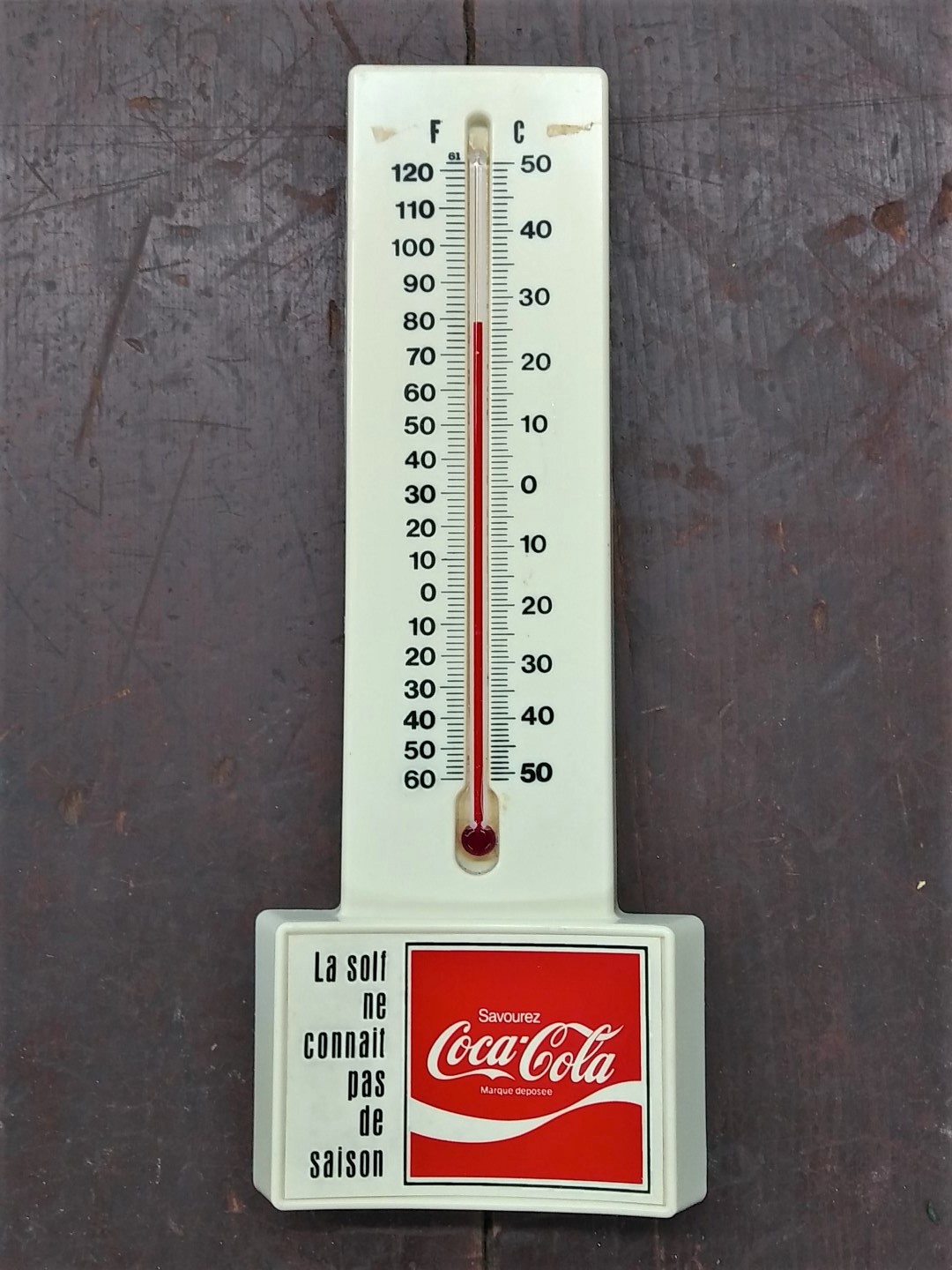The image depicts a worn gravestone floor that is heavily scratched and marked. At the very center of this gravestone, there is an unusual feature: a thermostat sponsored by Coca-Cola. 

The design elements on the thermostat include a vertical inscription on the left side which reads "L.A. S.O.L.F."; beneath that is "N.E."; followed by "C.O.N.N.A.I.T."; then "B.A.S."; "D.E."; and lastly "S.A.I.O.S.O.N.". To the right, there's a prominent red square incorporating a white river-like stripe running through it. Above this square, the text "Coca-Cola" is displayed, with the term "S.A.V.O.R.U.R.E.S.E." positioned above that.

The thermostat is divided into Fahrenheit on the left side and Celsius on the right side. The Fahrenheit scale ranges from 60 at the bottom to 120 at the top, while the Celsius scale ranges from -50 at the bottom to 50 at the top. A red dial at the center of the thermostat shows a liquid that measures up to 80.

Surrounding the thermostat is a black stripe encircling it. The bottom part of the thermostat features a distinctive, firm square component that appears to offer depth and grip. The entire fixture is a curious and detailed installation, contrasting sharply with the distressed gravestone floor.